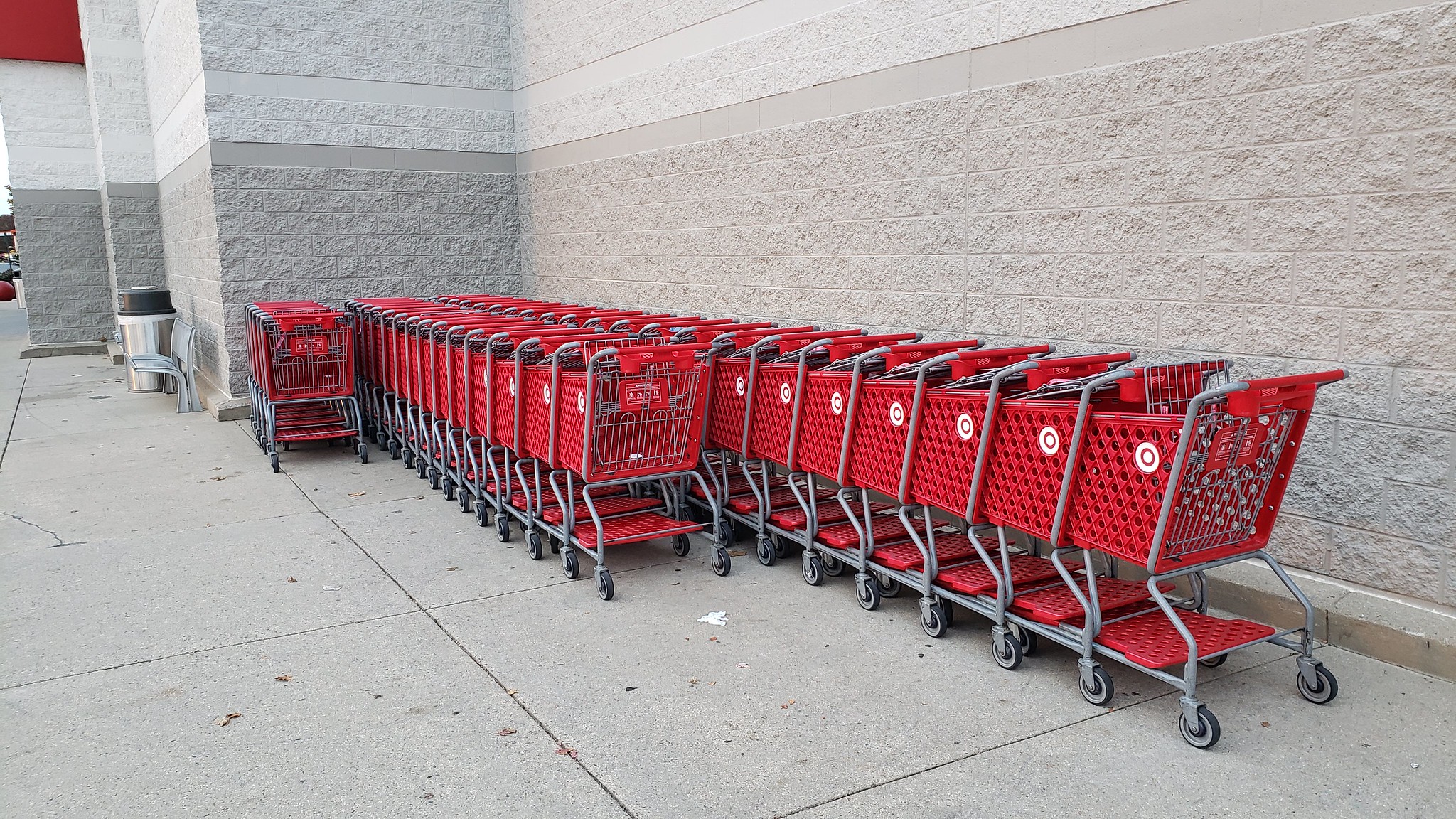This photograph captures the exterior of a Target store with distinct architectural details, notably the concrete block walls that are gray in color and the white upper sections. Dominating the scene are three rows of the store's signature red shopping carts, each featuring the iconic white and red bullseye logo near the handle. The shopping carts are neatly nested within their respective rows, which vary in length. On the left, the shortest row consists of approximately five carts, while the middle row has a moderate number. The rightmost row is the longest, with a sizeable collection of carts parked against the Target wall. The gray pavement of the parking lot underscores the vibrant red of the carts, creating a striking visual contrast. Additionally, the upper left-hand side of the image reveals the entrance of the store, completing the composition of this well-organized and descriptive photograph.